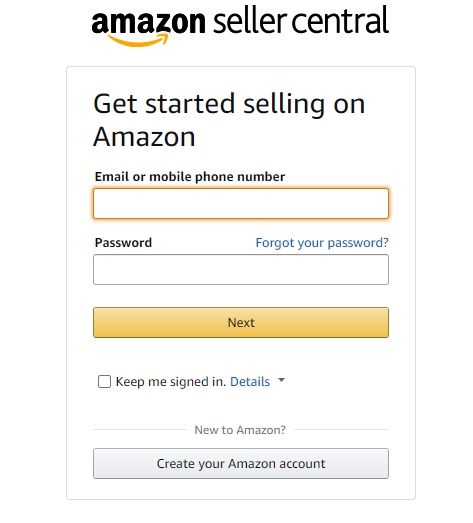The image depicts the Amazon Seller Central login page with the following elements arranged on a white background:

1. **Header**:
   - **Text**: "Amazon Seller Central"
   - **Location**: At the top of the page.

2. **Login Prompt**:
   - **Text**: "Get started selling on Amazon"
   - **Location**: Below the header.

3. **Email or Mobile Phone Number Field**:
   - **Description**: 
     - A data entry field with a black outline and a faint yellow/golden glow.
   - **Placeholder**: "Email or mobile phone number".

4. **Password Field**:
   - **Description**: 
     - A white data entry field with a gray outline.
     - To the right, in blue text with a question mark: "Forgot your password?"

5. **Next Button**:
   - **Description**: 
     - A yellow-orange button with a black or gray outline, the same size as the email and password fields.
     - Text on the button: "Next".

6. **“Keep me signed in” Checkbox**:
   - **Description**: 
     - A small square with an unchecked checkbox.
   - **Details**: "Details" with a blue drop-down indicator.

7. **New to Amazon?**:
   - **Text**: "New to Amazon?"
   - **Style**: In gray, flanked by gray lines on either side.

8. **Create Your Amazon Account Button**:
   - **Description**: 
     - A gray button with a gray outline, the same size as the data fields and the "Next" button.
     - Text on the button: "Create your Amazon account".

**Color Scheme**:
- Predominantly white background.
- Text colors include black, gray, and blue.
- Button colors include yellow-orange and gray.